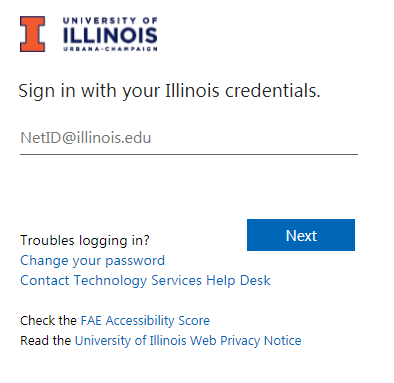This vertical image prominently features a login screen for the University of Illinois. At the top, there is an orange eye icon outlined in blue. To the right of the icon, it reads "UNIVERSITY OF" in blue, all capital letters with a smaller font size. Below, "ILLINOIS" appears in larger, blue, all capital letters. Beneath "ILLINOIS," in the smallest font size and still in all caps, it states "URBANA-CHAMPAIGN."

Further down, the text "Sign in with your Illinois credentials" is written in black font. Below this, there is a black line followed by instructions that read: "NetID" (with "ID" capitalized), the "@" symbol, and "illinois.edu." 

To the right of this, there is a horizontal, rectangular area with a turquoise background. Inside it, "NEXT" is written in white, bold font. On the left side of the turquoise area, "Trouble logging in?" is written in standard font. Below that, in blue font, it says "Change your password," followed by "Contact Technology Services Help Desk" on the next line.

There is a space, then the text "Check the FAE accessibility score" appears, with "FAE" in blue, all caps font and the rest in black font. Following this, "Read the" is written in black font on the next line, and immediately below, "University of Illinois Web Privacy Notice" is in blue font.